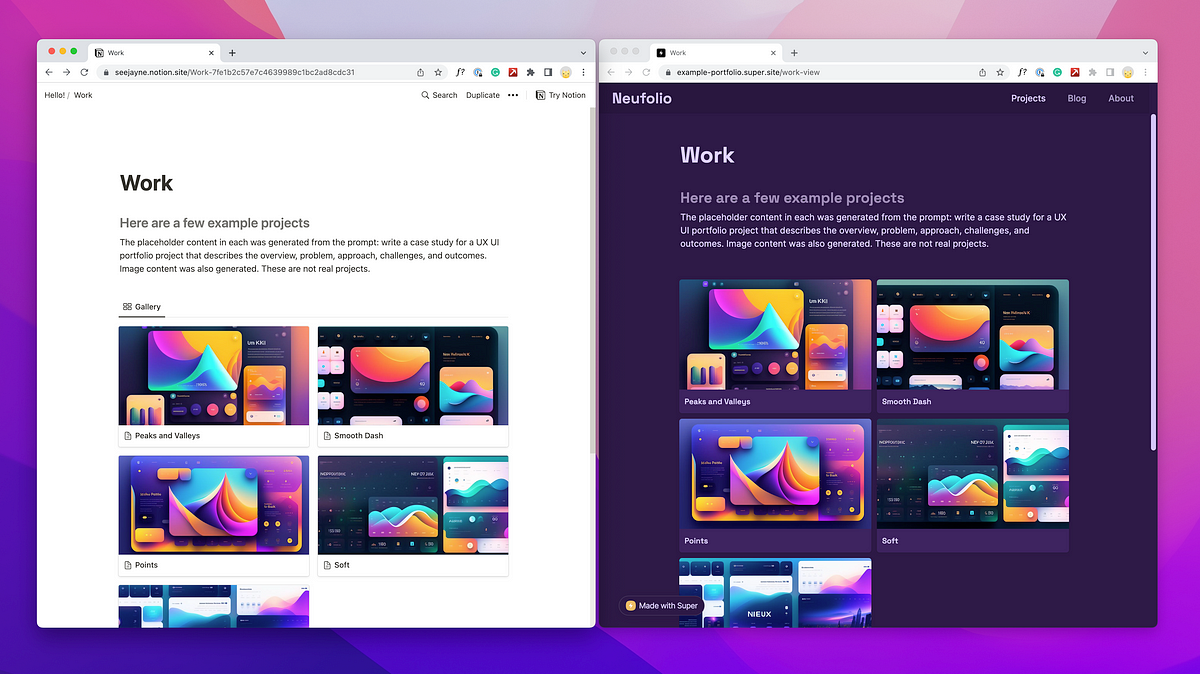The image features a dual-monitor computer setup, with two screens placed side-by-side. The background gradient transitions from pink, purple, and navy to hints of lavender and peach at the top, creating a visually vibrant backdrop.

On the left screen, the background is white, displaying a workspace titled "Work." This section includes several example projects, each a product of a prompt designed to simulate a UX/UI portfolio case study. The prompt instructed the generation of an overview, problem, approach, challenges, and outcomes, emphasizing that the projects and images are entirely fictional. The screen showcases an arrangement of project titles including "Peaks and Valleys," "Smooth Dash," "Points," and "Soft."

The right screen contrasts with a dark navy or black background, also titled "Work," matching the example project structure found on the left. The prompts here are similarly described, directing the creation of case studies with placeholder content. The accompanying generated images are labeled "Peaks and Valleys," "Smooth Dash," "Points," "Soft," and an additional part of the content that appears to be cut off at the bottom.

This detailed caption captures the essence and structure of the workspace setup, highlighting the use of generated content for illustrative purposes.